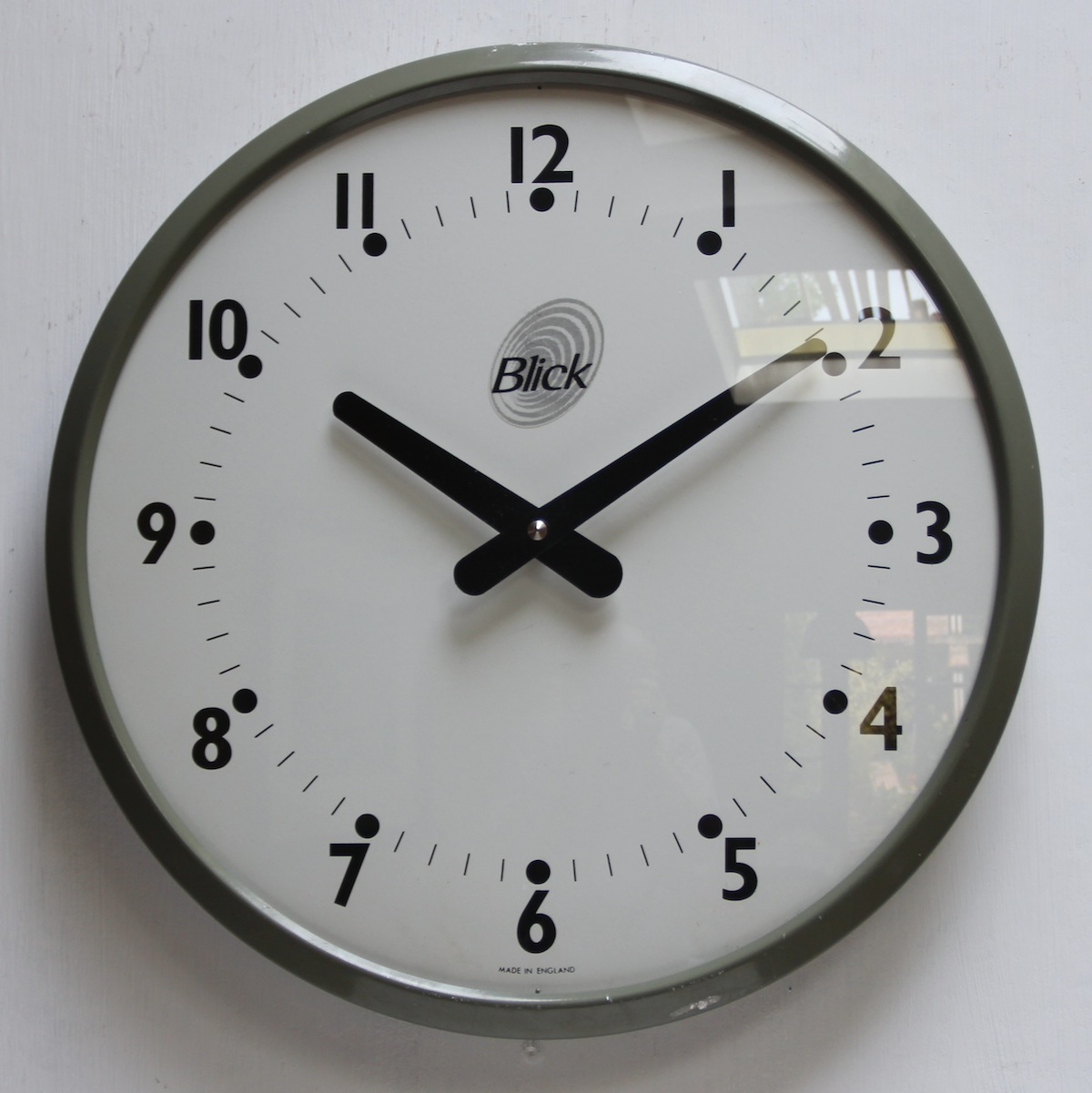The photograph prominently features a circular clock with a strikingly simple and modern design. The clock is framed in a dark grey borderline, casting a subtle shadow on the light gray background. The clock face is bright white, overlaid with black numerals from 1 to 12, each accompanied by a small black dot at their base. Positioned at the top beneath the number 12, there's a logo that reads "BLICK," accompanied by a swirl of grey circles angled to the right. The clock's black hands are set to a time indicating the short hand at 10 and the long hand at 2. Notably, there are reflections of a possible window visible on the numbers 2 and 4, suggesting light interplay captured in the photograph. At the bottom beneath the number 6, there is a line of text too small to discern. This clock, hanging against the wall, evokes a minimalist and functional aesthetic.